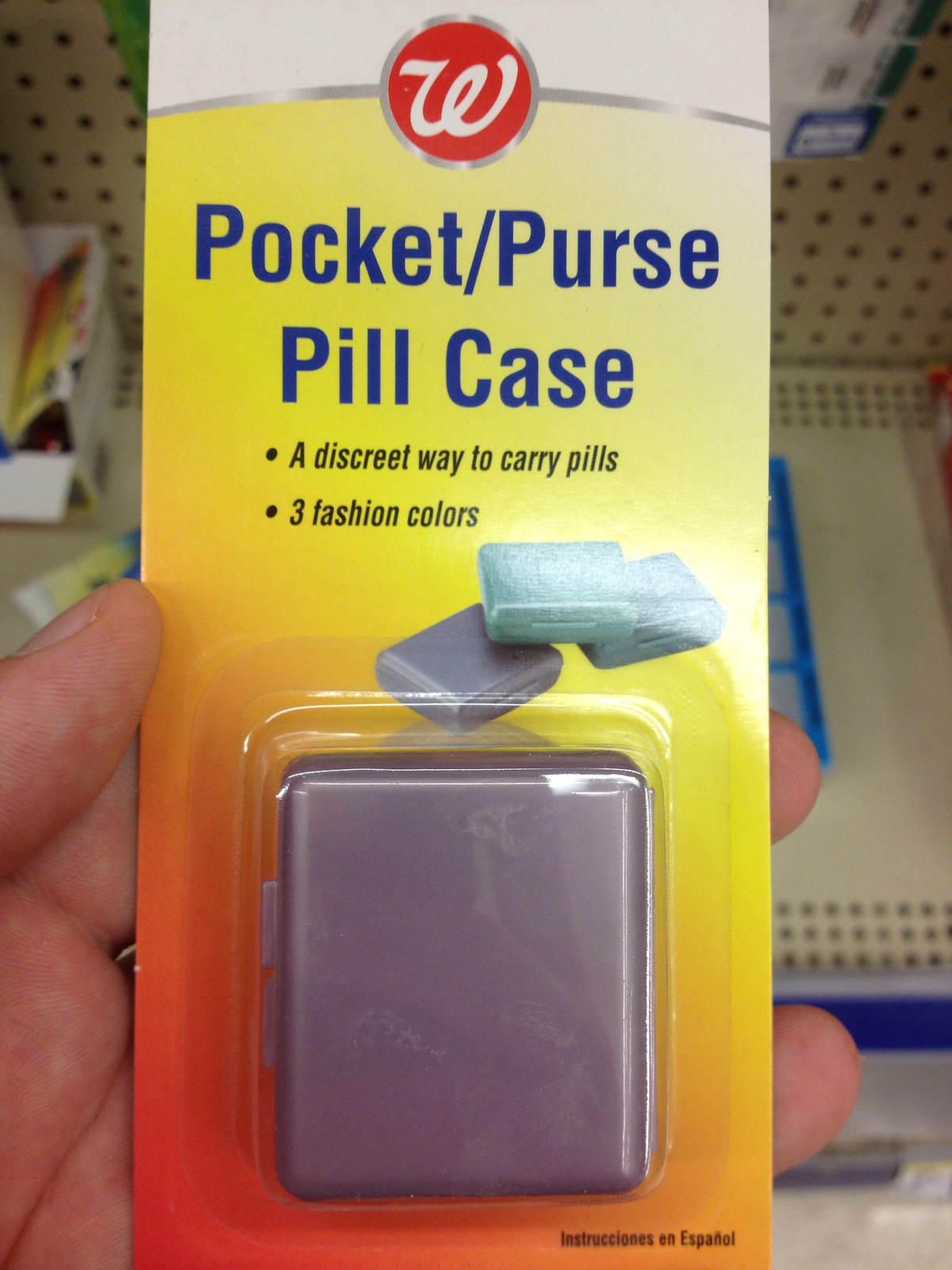In this photo, a person's hand, emerging from the lower left and grasping the item with their thumb on the left edge and fingertips supporting it from behind, displays a Walgreens brand pocket purse pill case. This product, designed as a discreet way to carry pills, is packaged and prominently features its claim of coming in "three fashion colors". The packaging transitions from a light yellow to a deep orangey-red background and includes navy blue writing. The packaging shows three available colors: purple, light blue, and darker blue, with the person specifically holding the purple one. Additional details include a mention of instructions in Spanish and a silver banner framing the Walgreens logo at the top. The background reveals store shelves, emphasizing the retail setting, with another type of pill case visible hanging on the shelf in the top right corner.